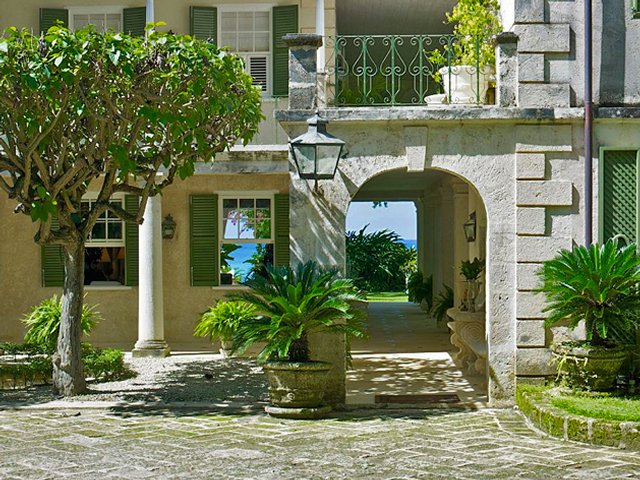This color photograph captures the facade of a high-end residence, potentially a historic southern-style home or an upscale apartment complex. The scene is set outdoors, showcasing a large entryway flanked by a concrete archway, giving way to a walkway beneath a covered stairway. The structure predominantly features stone-textured or stucco walls with large corner-style bricks, adorned with white, green-shuttered windows on both floors.

In front of the archway, a couple of slightly dirty, greenish potted plants are placed, while a freshly pruned tree stands to the left. The stairway leads up to a balcony marked by a green wrought iron railing, where more potted plants, including a prettily painted white pot, are arranged. You can spot an air conditioner unit in one of the windows above.

The exterior also includes some distinctive elements: a white brick driveway with moss-covered patches indicating the building's age, a few pillars defining the entryway, and a zigzag pattern of paving stones surrounded by lush greenery. To the right, a medium-sized pruned tree complements the verdant scene, which hints at a costal or lakeside location, as glimpses of water are visible through the archway and one of the lower windows. Additionally, an external lantern extends from the wall near the entrance, enhancing the sophisticated charm of the property.